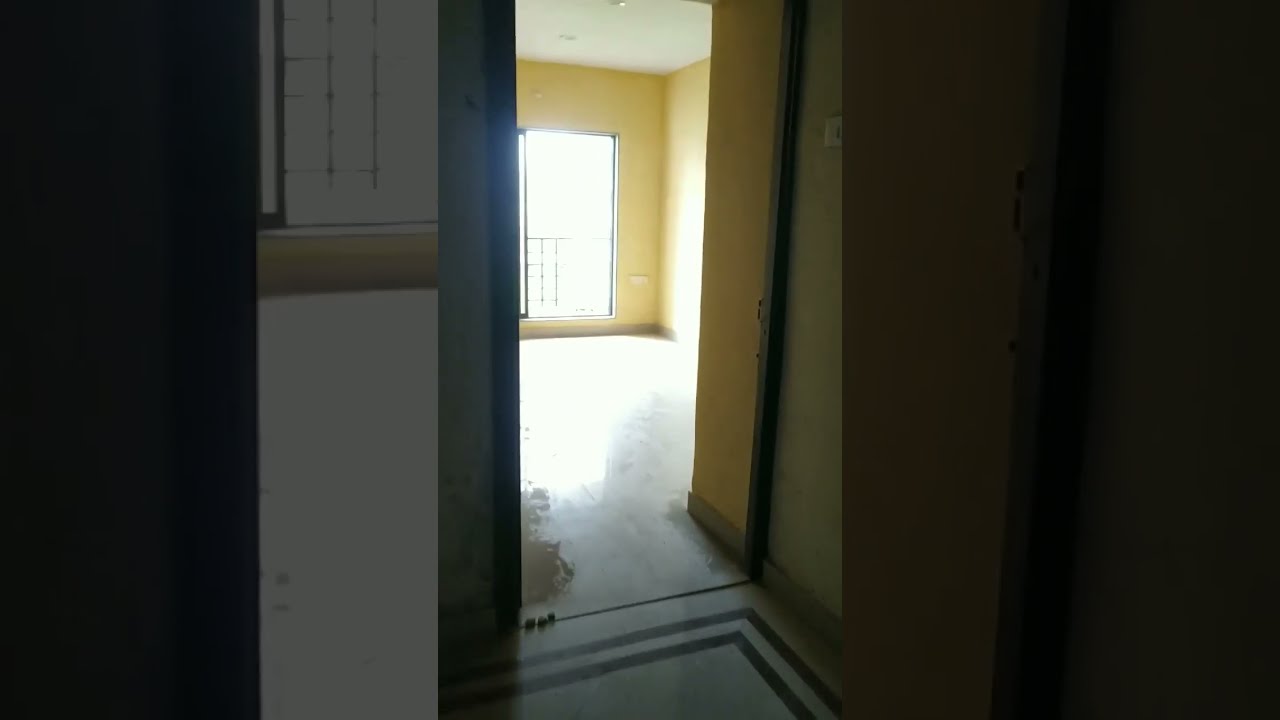The photograph captures the interior of a dark, unfurnished house viewed from a hallway. It is taken from the perspective of the hallway looking into a brightly lit room with a large sliding glass door or window at the far end, through which intense natural light floods in, creating a stark contrast against the dim hallway. The walls in the illuminated room are a deep golden yellow, featuring a brownish border edging at the bottom, while the ceiling is white. The floor appears to be light-colored tile, possibly linoleum, with a couple of black pinstripe designs on the outer edges. Just outside the threshold of this room, on the hallway's right wall, a thermostat is visible. The lighting in the photograph is very poor, enhancing the gloomy atmosphere within the darker part of the house, while the bright white light from outside accentuates shadows and defines the empty space within the room.